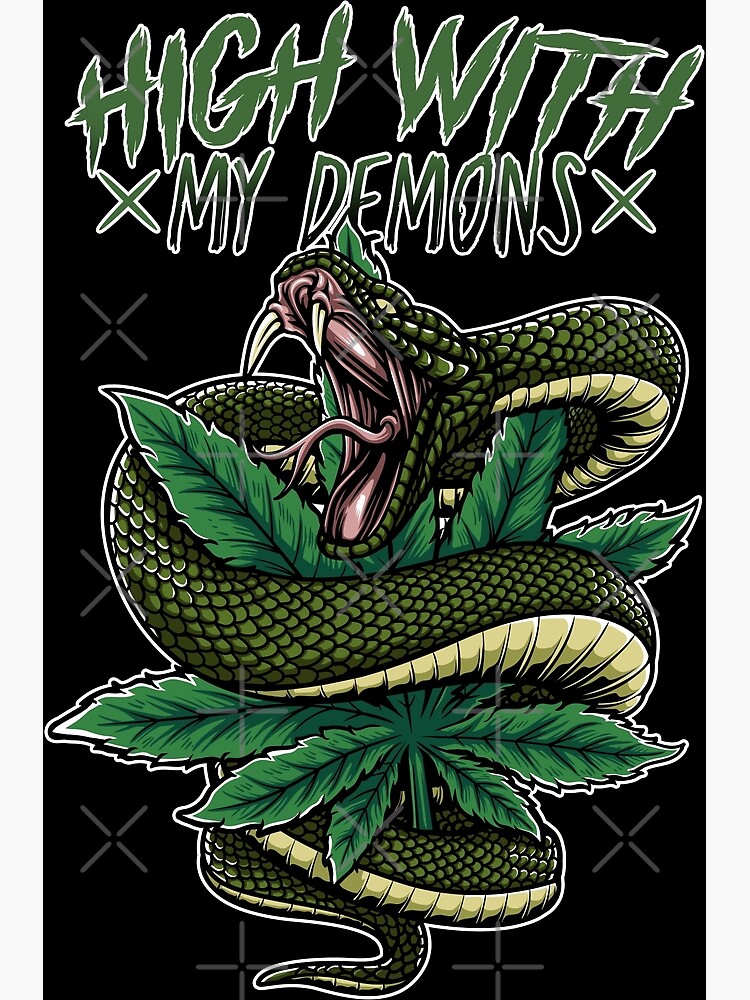The image is a computer-generated graphic art with a black background, displaying a vivid illustration of an angry, cartoon-style snake with huge fangs and a pink mouth. The snake, featuring a bumpy texture like an alligator and colored in various shades of green—including a warmer pea-colored top and a lighter green belly—is prominently wrapped around a bright green marijuana leaf. The composition is further accentuated with green text reading "Hi with my demons," where "my" and "demons" are framed by green X's. Similar X-shaped symbols are dispersed as watermarks across the artwork, adding to the distinctive visual texture.